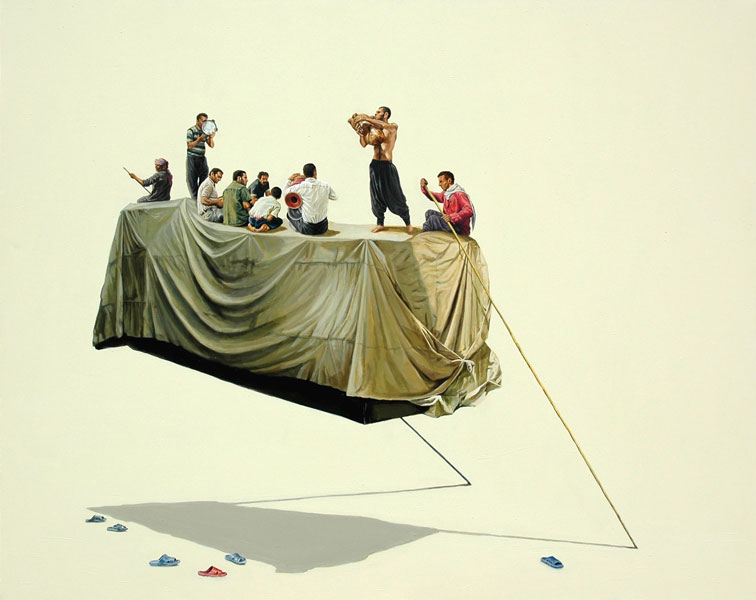The painting depicts a surreal scene with a cream background. A large, rectangular platform covered in a gold or cream-colored cloth is suspended in mid-air, seemingly held up by thin, nearly invisible wires. Surrounding this floating platform are the shadows cast onto the cream surroundings, emphasizing the illusion of flight. 

On the platform, which resembles stacked crates beneath the cloth, sits a group of nine men. At the back, a man in a red, long-sleeve shirt wields a long pole reminiscent of a gondolier's oar, creating an intriguing contrast with the lack of visible ground. Beside him, a shirtless man in black balloon pants stands prominently, playing a saxophone-like instrument. Nearby, a seated man in a long-sleeve white shirt and dark pants is joined by another person displaying only their back, clad in a white shirt and dark pants, appearing smaller and younger. 

Towards the left side of the platform, another figure in a green shirt can be seen amidst the seated men. At the front, a shirtless man blows into a saxophone-like instrument while standing confidently. Scattered blue and red flip-flops on the platform add subtle splashes of color to the primarily cream and dark-toned scene. The overall composition blends elements of realism and fantasy, inviting endless interpretation.